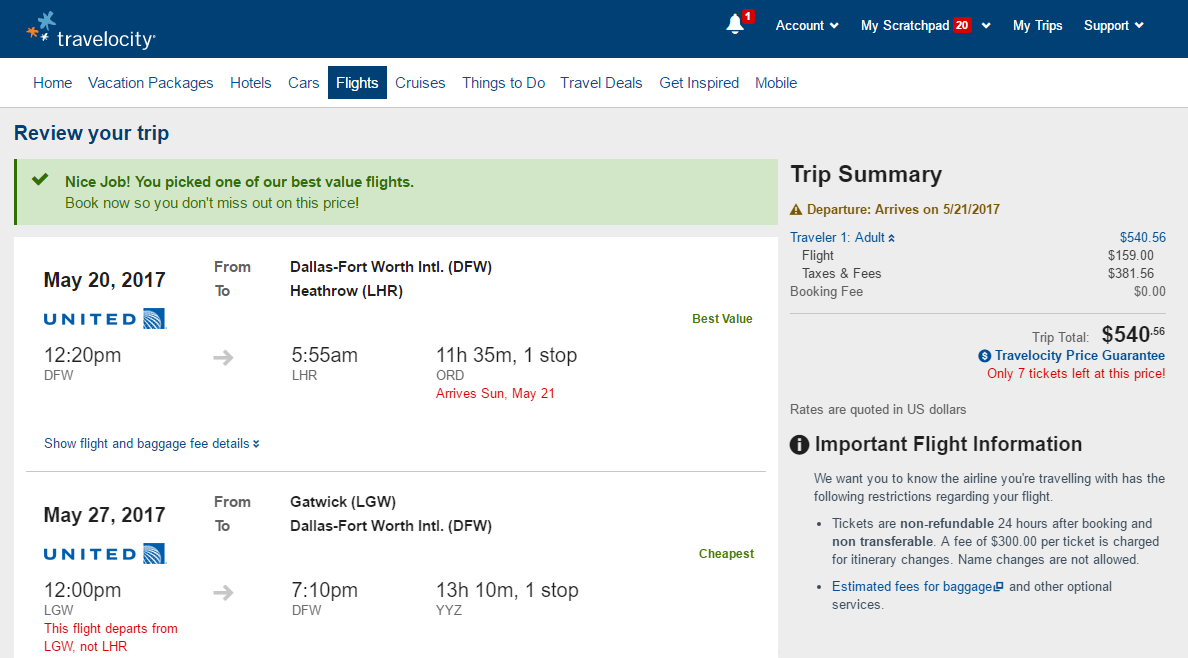This is a detailed caption for an image from the Travelocity website:

---

The image displays a page from the Travelocity website. At the top left corner, the word "Travelocity" is prominently featured in white text. Next to the brand name is a logo comprised of oblong shapes in blue, orange, and white. Adjacent to the logo, there is a white bell icon with a red notification badge indicating the number "1".

To the right of this section, a red box with the number "20" highlights the "Scratchpad” function. Additionally, the top menu bar includes links labeled "My Trips" and "Support".

Below this header, a navigation menu lists various tabs: "Home," "Vacation Packages," "Hotels," "Cars," "Flights" (highlighted in a blue box), "Cruises," "Things To Do," "Travel Deals," "Get Inspired," and "Mobile."

Further down, a blue text heading reads "Review Your Trip," followed by a green notification stating, "Nice job! You picked one of our best value flights. Book now so you don't miss out on this price."

The main body of the page displays flight details for a trip. The first flight listed is on May 20, 2017, with United Airlines, departing from Dallas Fort Worth International (DFW) at 12:20 p.m. and arriving at Heathrow at 5:55 a.m. the next day. The total travel time is 11 hours 35 minutes with one stop at ORD (Chicago O'Hare International), arriving on Sunday, May 21.

The return flight is shown below, with a departure date of May 27, 2017. On the right side of the page, a "Trip Summary" section itemizes costs for the flight, taxes, and booking fees, totaling $540.56. Additionally, an "Important Flight Information" note mentions that tickets are non-refundable.

---

This caption provides a thorough and structured description of the Travelocity booking page as depicted in the image.